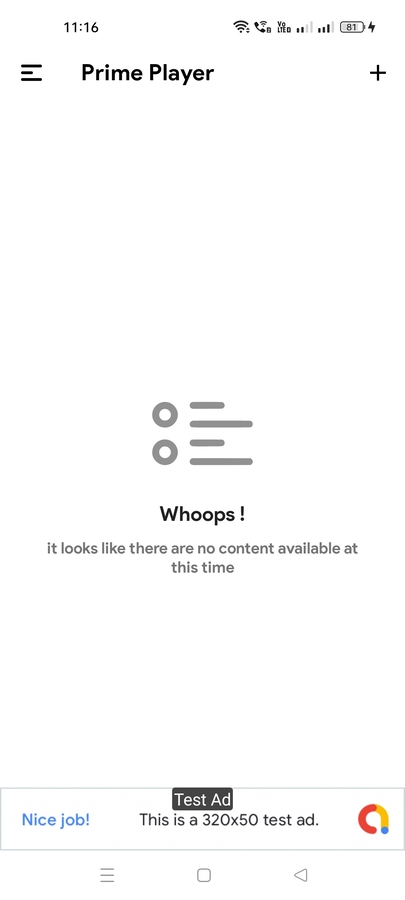The screen of a mobile device displays various information:

At the top, against a white background, the time is indicated as 11:16 on the left. In bold text below, 'Prime Player' is displayed above three black lines. To the right, there is a bold plus sign. Above this, the Wi-Fi icon shows full bars, indicating excellent reception. Adjacent to it, a black phone icon is visible, next to the text 'Rio LTED?'. The reception shows two out of four bars, and another indicator shows three out of four black bars. A black lightning bolt icon signifies that the phone is charging, currently at 81%.

At the bottom, there are four gray lines with two gray circles on the left. Below this, the text 'Whoops!' is in black, followed by a gray message: 'It looks like there are no content available at this time.' Further down, a rectangular gray-outlined box contains two buttons. To the left, a white and blue button exclaims 'Nice Job!'. In the middle, a gray rectangular button with white text reads 'Test Ad'. Below it in black text, 'This is a 320 x 50 test ad.' To the right of the text, a gradient 'A' transitions from red to yellow to blue.